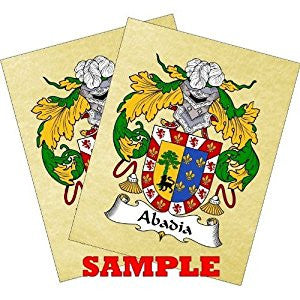The image showcases two small, rectangular, portrait-oriented pieces of paper or cards with an off-yellow background, stacked with one slightly tilted to the left and the other slightly to the right. Both cards feature an elaborate coat of arms in the center. The shield at the center is divided into two halves: the left side is blue with yellow crowns and leaves, and the right side is yellow containing a green tree and a black lion. This intricate shield is framed by elaborate green and yellow leaves and filigree that drape around it. Below the shield is a decorative white ribbon with the word "ABADIA" inscribed on it in capital letters. At the very bottom of the cards, the word "SAMPLE" is stamped across both in bold red capital letters. The visual creates a vivid heraldic design with rich colors including reds, blues, greens, and yellows.